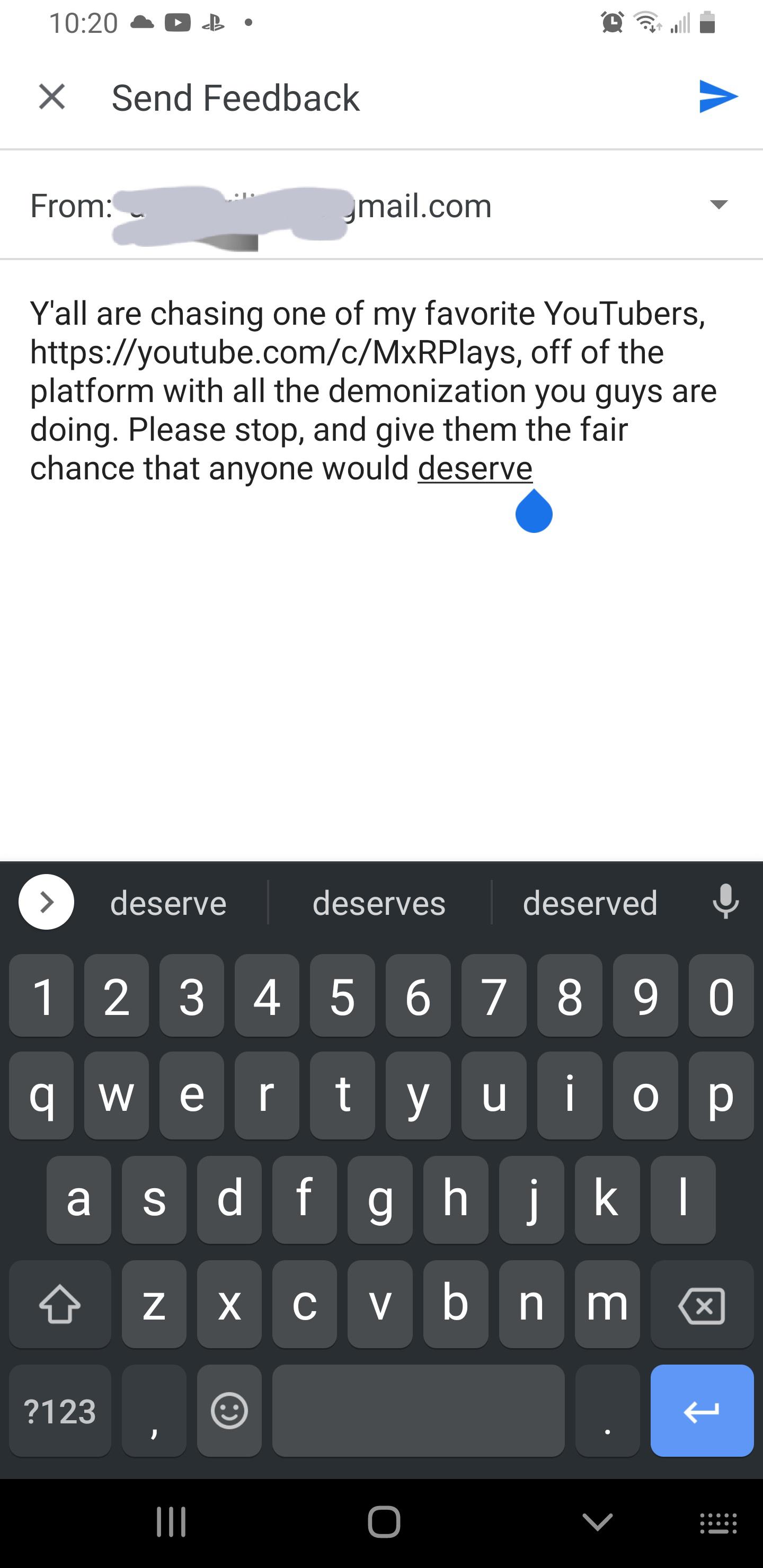The image is a screenshot taken from a cell phone, displaying a feedback form. At the top of the screen, the title "Send Feedback" is visible. To the right of the title, there is a blue send arrow icon.

Below the title, there is a "From" section. The email address begins with redacted characters and ends with "@gmail.com." Adjacent to this email address is a dropdown arrow.

The main content of the feedback form follows, where the user has typed a message: 
"y'all are chasing one of my favorite YouTubers, https://youtube.com/c/mxrplays. This is off of the platform with all the demonetization you guys are doing. Please stop and give them the fair chance that anyone would deserve."

At the bottom of the screen, the cell phone's keyboard is visible, indicating that the user is in the process of typing. The status bar of the phone shows the time as 10:20, and the phone has two bars of signal reception.